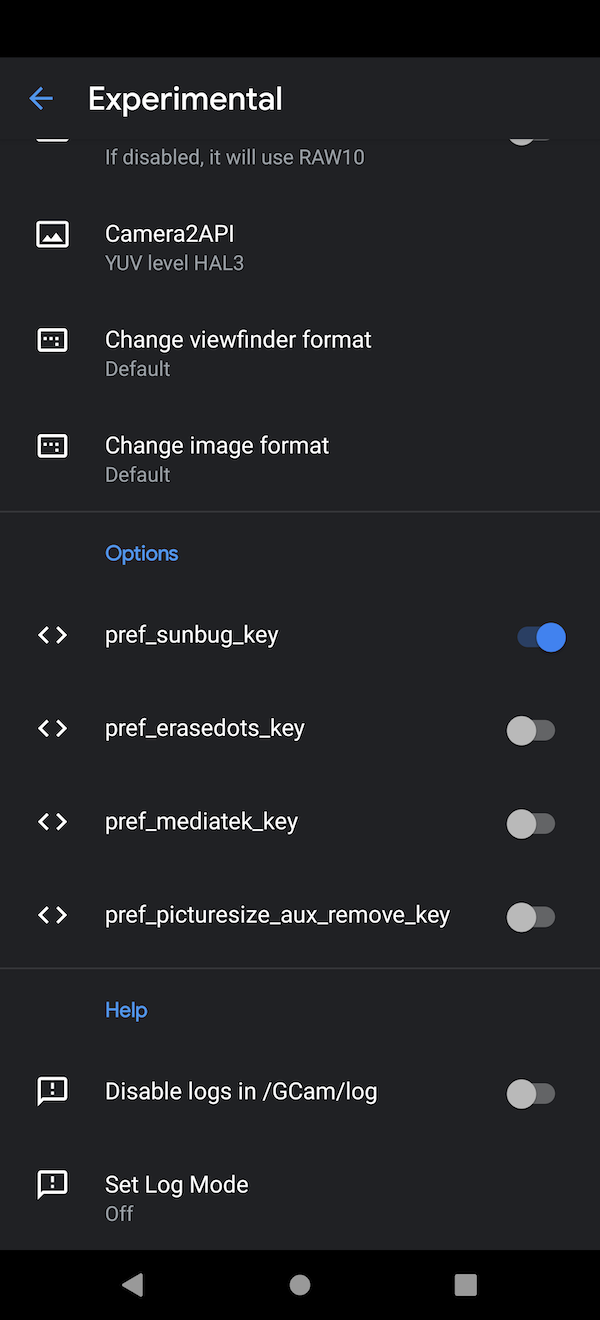This image is a vertical screenshot taken on a mobile phone, showcasing what appears to be an experimental settings menu for a camera application. 

At the top of the screen, there is a horizontal black box followed by a dark gray background. The word "Experimental" is prominently displayed in white text at the top. Below it, a sentence reads, "If disabled, it will use RAW 10."

The following options are listed:
- **Camera 2 API:** YUV level, HAL 3 (accompanied by an icon resembling a photograph).
- **Change viewfinder format:** Default (with an icon that looks like a rectangle with three horizontal dots and one dot underneath the third horizontal dot).
- **Change image format:** Default (with the same icon).

Further down, a blue hyperlink labeled **"Options"** appears, leading to additional settings:
- **pref_sunbug_key:** Toggle switched on.
- **pref_erase_dots_key:** Toggle switched off.
- **pref_mediateK_key:** Toggle switched off.
- **pref_picture_size_ox_remove_key:** Toggle switched off.
- **Help:**
  - **Disable logs in /GCAM/log:** Toggle switched off.
  - **Set log mode:** Off.

This screenshot seems to provide a comprehensive view of the camera app's experimental settings, detailing various toggled options and their current statuses.